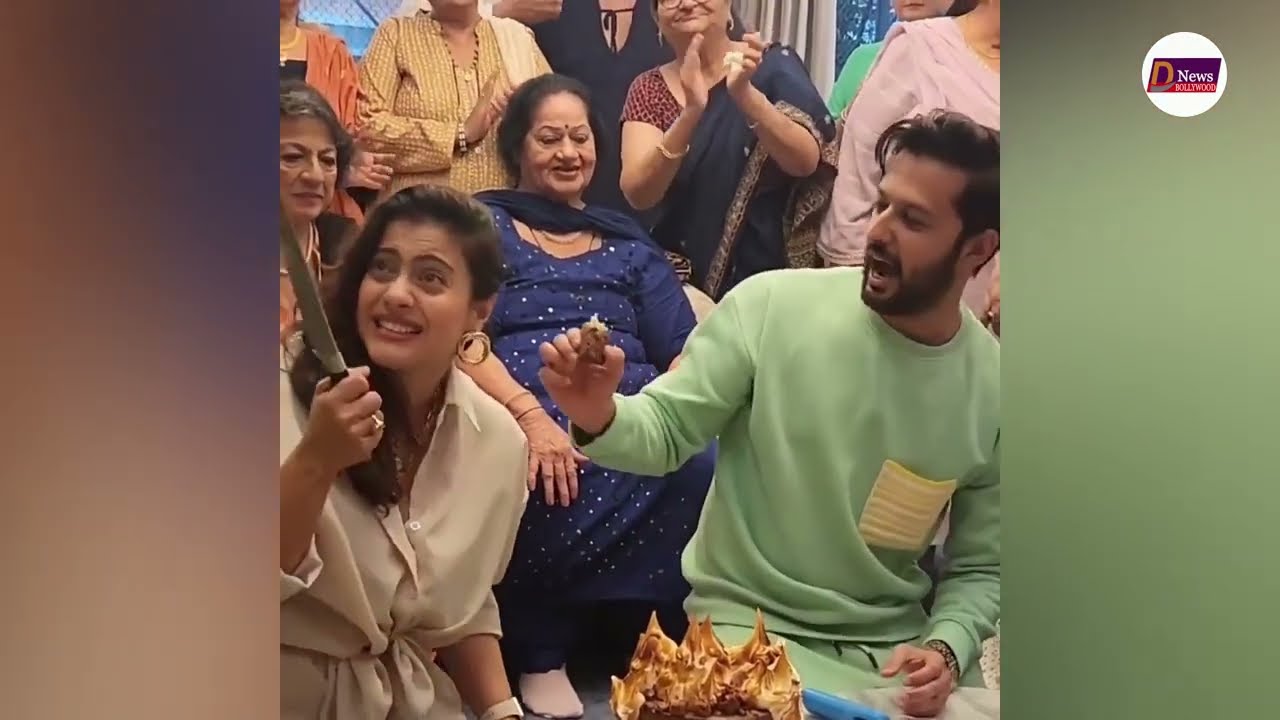The central focus of the image is a lively scene featuring a group of South Asian individuals, with the foreground dominated by a young woman and a young man. The woman, likely in her thirties, has braided gold hoop earrings, a gold ring, and a somewhat tense expression. She's holding a large, silvery butcher knife. Her attire includes a khaki-colored silk top with a collar and an off-white belt. On her right, a bearded young man with medium-length brown hair and a green sweatshirt with a distinctive yellow pocket holds a piece of food, possibly fruit or a piece of fruitcake, looking surprised and engaged with the woman.

The background showcases several other South Asian people, some sitting and appearing to enjoy what seems to be a festive or celebratory event. Notable among them is an elderly woman in a navy blue sari, distinctive with a maroon bindi on her forehead. Others are seen smiling, clapping, or paying attention to different facets of the gathering.

The image composition includes blurred quarter segments on the left and right edges, filled with gradient colors—browns on the left and greens on the right—framing the central action. The top right corner also features a small, gold "D" inside a white circle next to the word "news" in white text.